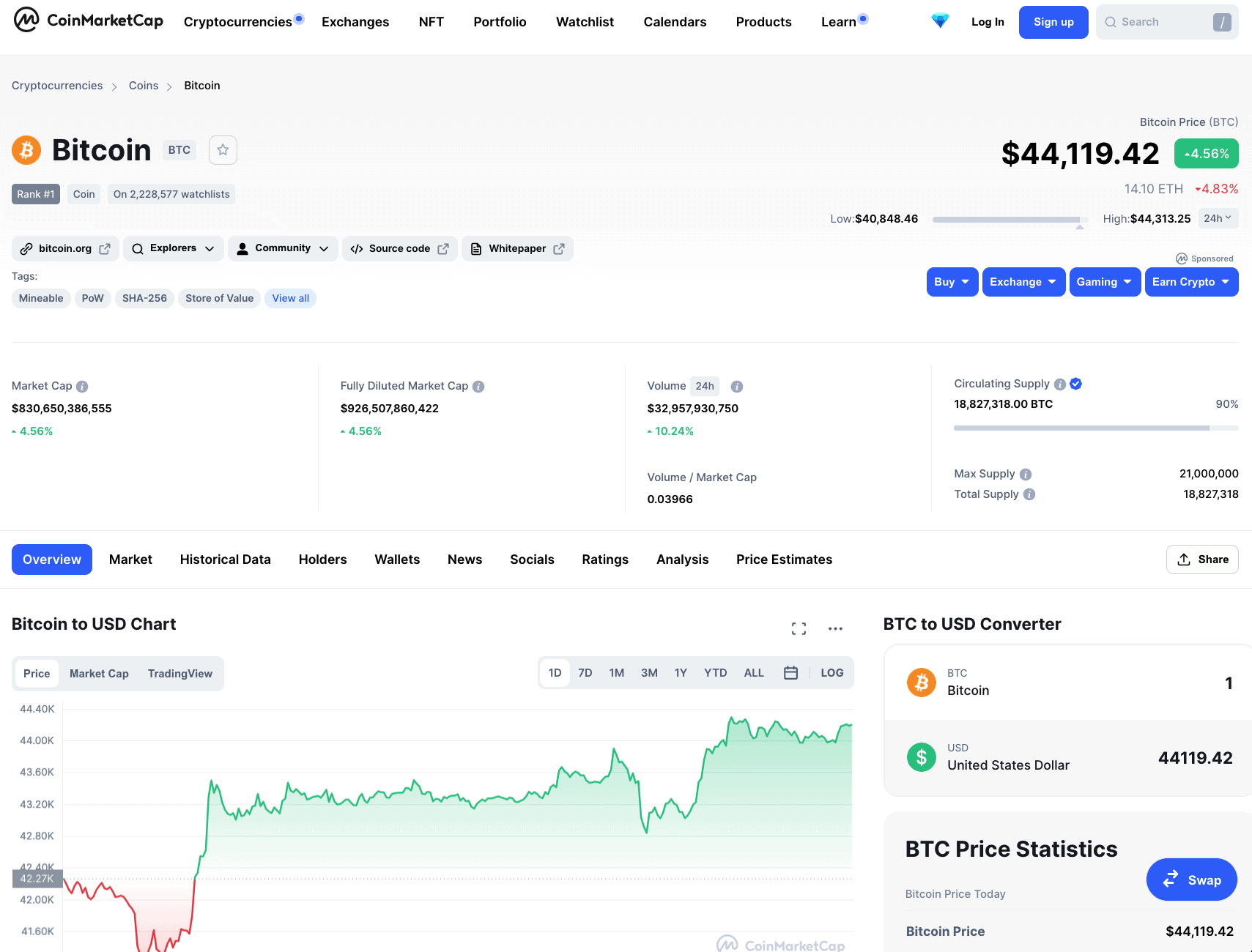This is a detailed description of a screenshot from the CoinMarketCap website, specifically the Bitcoin page. 

The interface includes various navigation tabs at the top such as Cryptocurrencies, Exchanges, NFT, Portfolio, Watchlist, Calendars, Products, Learn, Login, and Sign-Up, with the Sign-Up button highlighted in blue. There is a search field for quick access to data. 

Currently, Bitcoin is selected, displaying that it is ranked number one. The main section shows the Bitcoin logo and has an array of financial metrics, including market cap, fully diluted market cap, and 24-hour trading volume. Notably, the 24-hour trading volume is approximately $33 billion.

Below these metrics, there's a trading chart providing a visual representation of Bitcoin’s price movements. Additional navigation options such as Overview, Market, Historical Data, Holders, Wallets, News, Socials, Ratings, Analysis, Price Estimates, and various timeframes for price fluctuation graphs are present.

The graph itself includes timeframes like 1 Day, 7 Day, 1 Month, 3 Month, 1 Year, and Year to Date, with green lines representing upward trends and a red line indicating a target price below the current trading price. To the right of the graph, the current Bitcoin price is listed as $44,119.42. 

Other elements visible include supplemental charts, a Bitcoin to U.S. Dollars converter, and detailed Bitcoin statistics at the bottom of the page. This comprehensive layout ensures users have access to all necessary data regarding Bitcoin's market performance and related analytics.